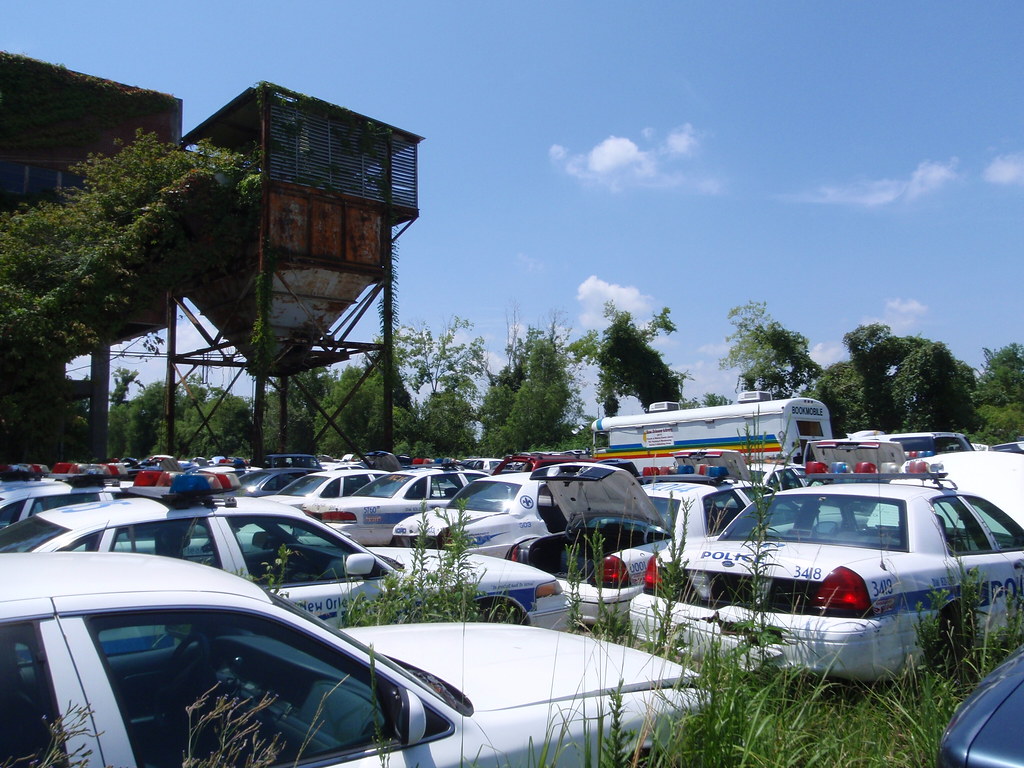In this image, abandoned police cars are scattered across a field of tall weeds and grasses, with a line of trees forming the background. There are approximately five or six police cars, primarily white with blue markings, and some with additional red and white lights. One of the police cars on the near right has "348" painted on it. Some of the cars have New Orleans written on them. The siren lights on top of the vehicles are old, pulsating red, white, and blue lights. Amidst the cars, there's a large bus-like vehicle labeled "Bookmobile," adorned with blue, green, yellow, and red stripes. To the left stands an old, rusty grain bin, approximately 35 to 40 feet tall. Additionally, there are two rusted brown and silver tanks. The sky is mostly clear, dotted with a few white clouds. No people are visible in the scene.